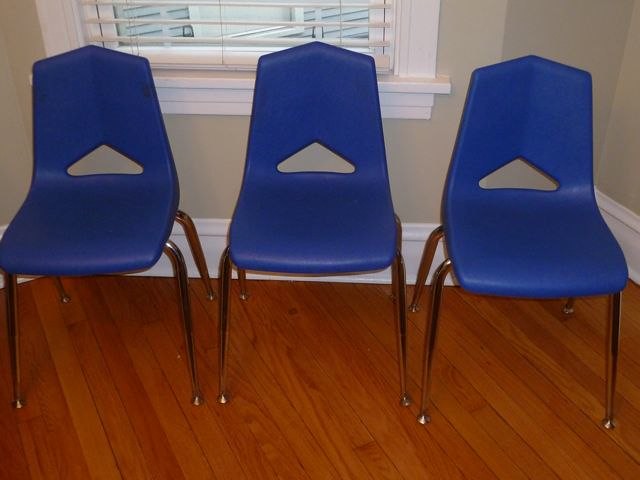This image depicts three identical blue plastic stacking chairs, characterized by their molded one-piece seat and backrest, which are a royal to navy blue color. Each chair has simple metal legs, described as having a gunmetal or cheap chrome appearance, and the backrests feature a small triangular cutout near the base, likely for ventilation or weight reduction. The chairs are positioned along a champagne-colored wall with white trim, situated against a window fitted with white louvered blinds, twisted open to allow light to filter through. Below the chairs is a medium brown hardwood floor. Notably, the room's corner is atypical, slanting backward at a 45-degree angle where the baseboards meet. The photograph appears to be taken from a slightly elevated angle, making the chairs and the area behind them the focal point of the image. Through the window, another window is visible, suggesting the camera's vantage point is from an elevated indoor position.